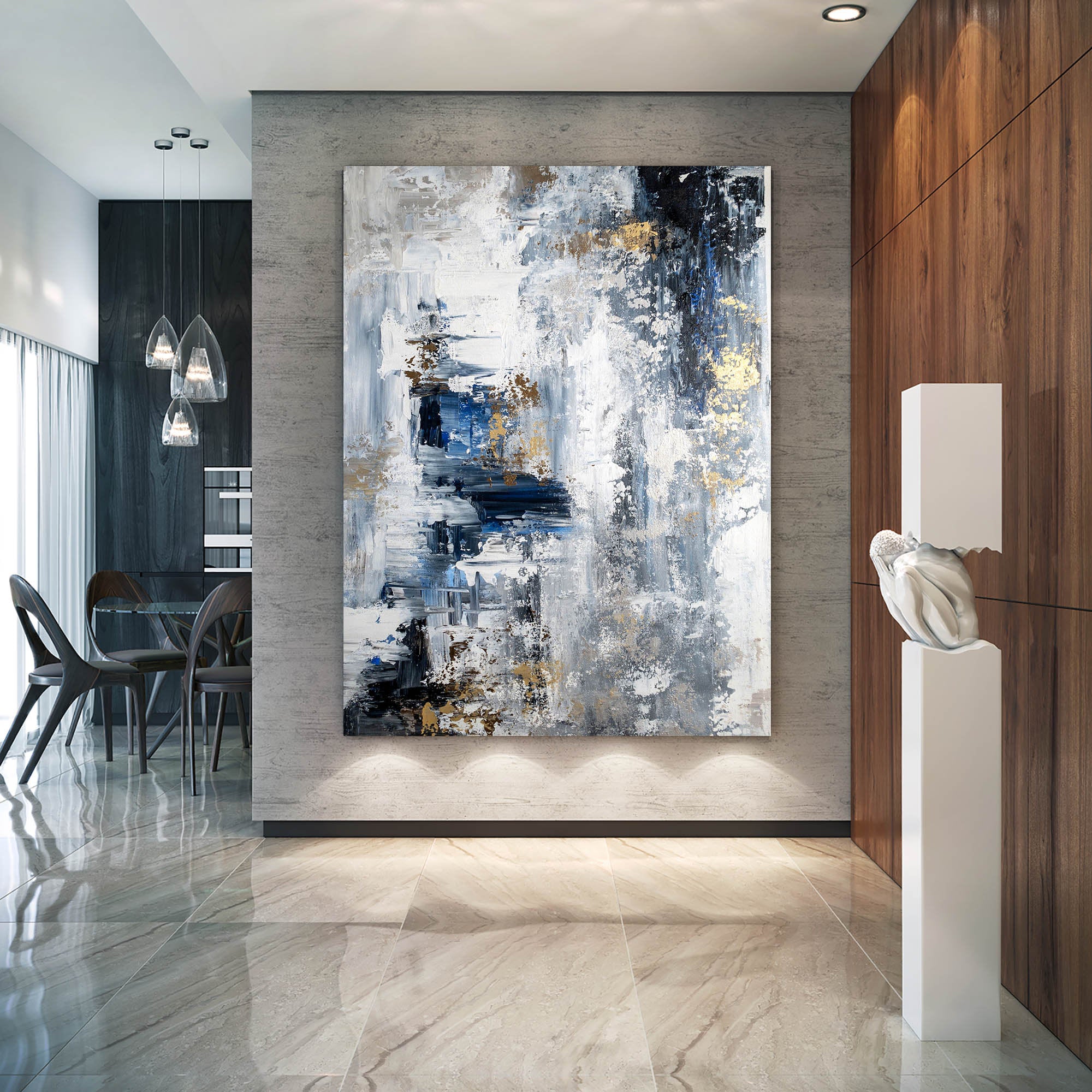The image captures a sophisticated interior, likely of a high-class home, showcasing an art-focused, contemporary aesthetic. The floor is composed of large, glossy marble tiles with white grout. Dominating the central wall of the main room is a striking, vertical contemporary wall hanging reminiscent of ice crystals, featuring horizontal and vertical lines in shades of blue and white, accented by splashes of gold. To the right, a darker wood-paneled wall is adorned with focused lighting, and in front of it stands an intriguing rectangular sculpture, intricately carved with a crouching human figure. This sculpture is described as white and positioned on a square stand. The room flows into an adjacent space where a sleek, modern kitchen set with a table, chairs, and pendant lights can be seen, continuing the luxurious and contemporary theme of the home.